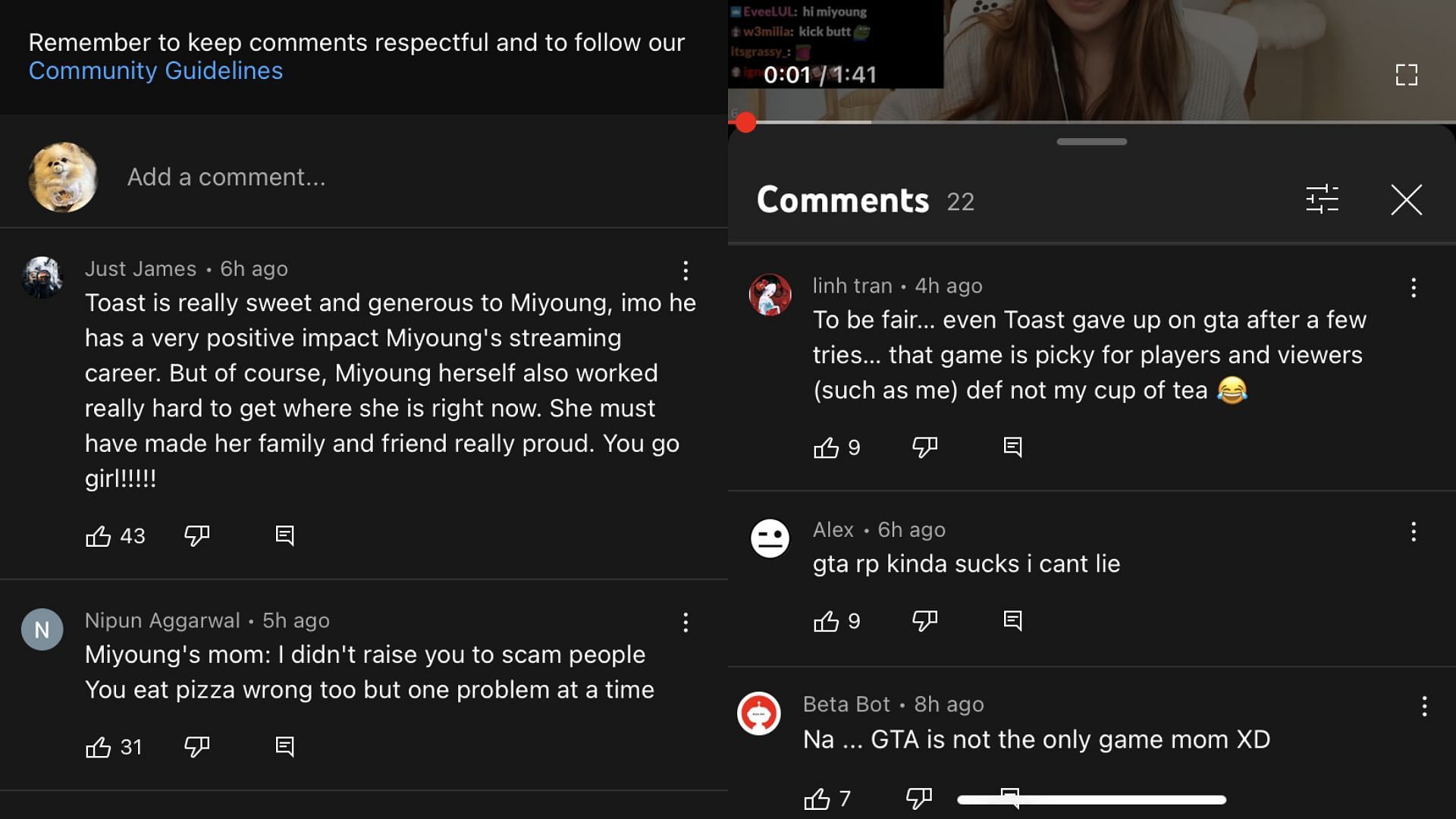This image is a screenshot from a website where users can comment on various topics. In the top left corner, there's a reminder for users to keep their comments respectful and to follow the community guidelines, with the phrase "Community guidelines" highlighted in blue. On the top right, there's a video in progress, featuring a woman with long hair, currently at 1 second into its 1 minute and 41 seconds duration, but the video is partially cut off.

Beneath the video, there are 22 comments displayed. Users are prompted to add their own comment next to a profile picture of a dog. Below this, we see several user comments. 

First, "Just James," who posted 6 hours ago, has a dog profile picture and commented, "Toast is really sweet and generous. In my opinion, he has had a very positive impact on my young streaming career. But, of course, me on herself also worked really hard to get where she is right now. She must have made her family and friend really proud. You go, girl." This comment has received 41 likes.

Next, "Nick Pond Agarwal" commented 5 hours ago, "Me along's mom, I didn't raise you to scam people. You eat pizza wrong too but one problem at a time." This comment has garnered 31 likes.

Another user, "Lynn Tron," posted 4 hours ago, "To be fair, even toast gave up on GTA after a few tries. The game is picky for players and viewers such as me, def not my cup of tea 😊." This comment has 9 likes, no dislikes, and no additional comments.

"Alex," who commented 6 hours ago, stated, "GTA RP kind of sucks I can't lie," and received 9 likes, with zero downvotes or comments.

Lastly, "Beta Bot" posted 8 hours ago, saying, "Now, GTA is not the only game for mom XD." This comment has 7 likes without any dislikes or additional comments.

A horizontal scroll bar is visible at the bottom of the comment section, positioned at the right.